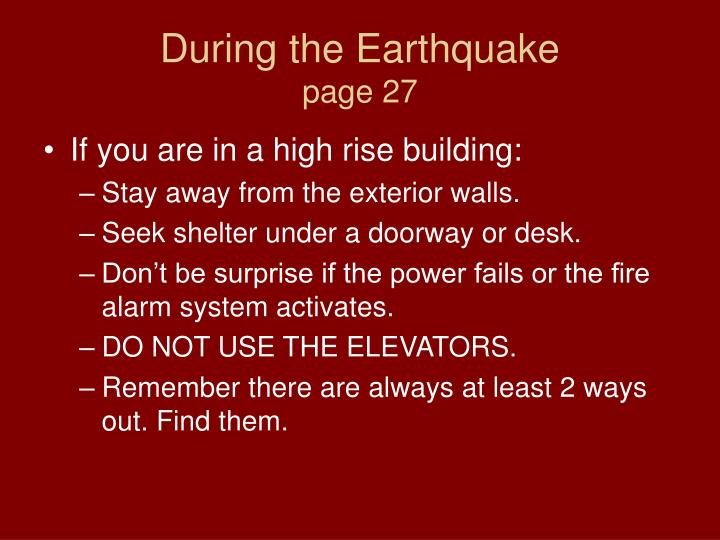The image is an informational slide with a solid dark crimson-red background. At the top center, in larger beige text, it reads, "During the Earthquake," followed by "Page 27." The text is predominantly white and styled as bullet points providing safety instructions for those in high-rise buildings. The points listed are: stay away from exterior walls, seek shelter under a doorway or desk, anticipate potential power failures or fire alarm activations, avoid using elevators, and remember that there are always at least two exit routes. The slide's overall appearance and formatting suggest it is part of a PowerPoint presentation.